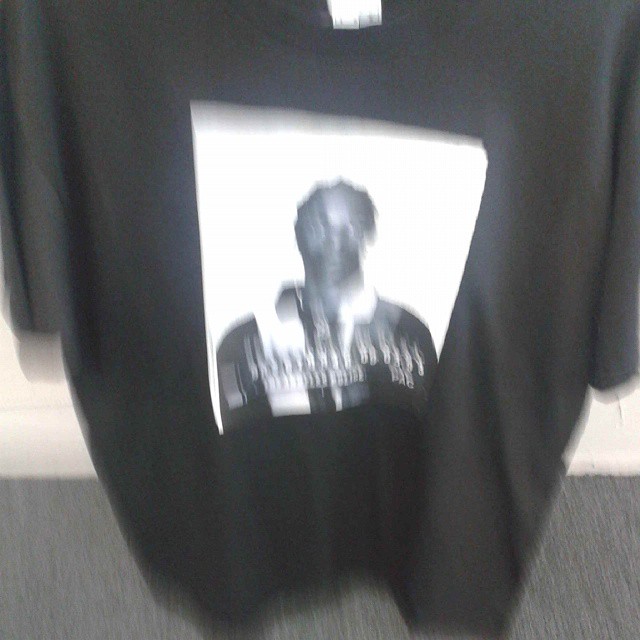The image features a black, short-sleeved t-shirt displayed against a light-colored wall and gray carpeting. The t-shirt has an iron-on patch in the middle, depicting a black and white mug shot of a black man wearing multiple jackets or coats. The mug shot, bordered by a white box, showcases the figure in various shades of grey, though the image is quite blurry. Vertical stripes can be seen on the man's attire, and numbers or some form of lettering appear at the bottom of the mug shot, though the text is illegible due to the image's blurriness. The tag of the t-shirt is visible near its collar.